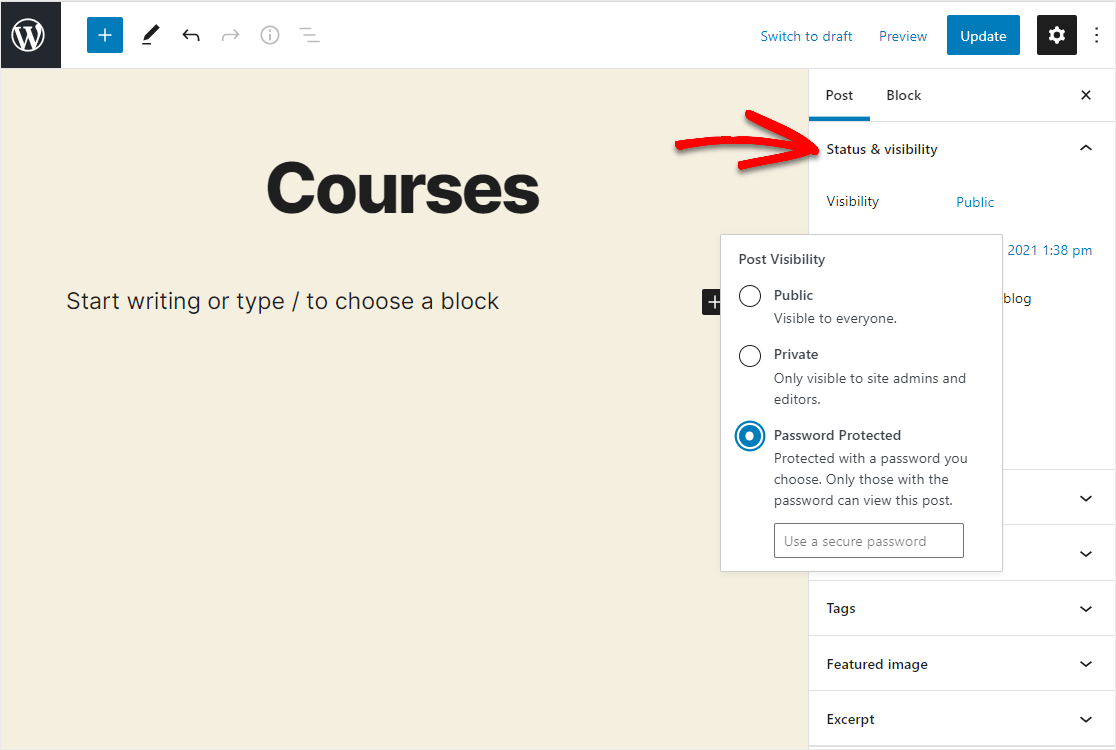This is a screenshot of the WordPress interface. In the top left corner, there is the WordPress logo, which is white against a black square background. Next to it is a white plus sign inside a blue box, followed by a pencil icon. Continuing to the right, there is a left arrow, a right arrow, an information symbol, and a three-line menu icon. 

On the top right, there is blue text reading "Switch to draft," followed by "Preview." Next to these options is a blue solid box with white text that reads "Update." Additionally, there is a black solid box containing a gear icon and a three-dot menu icon.

Beneath these elements, on the right side, the words "Post" and "Block" are displayed, with "Post" being highlighted by a blue line underneath it. To the right of "Block," there is an "X" icon.

Below this section, the "Status and Visibility" section is present with an upward arrow next to it. A red hand-drawn arrow is pointing to this section. Within this section, the word "Visibility" appears with the term "Public" mentioned below it. An adjacent box reads "Post Visibility." It includes three radio buttons: "Public," which is described as "Visible to everyone," followed by "Private," described as "Only visible to site admins and editors." The selected radio button is "Password Protected," which is described as "Protected with a password you choose. Only those with the password can view this post." 

Underneath this option, there is a white box with a black border that says "Use a secure password," accompanied by a downward arrow. Below this section, there are additional dropdown options titled "Tags," "Featured Image," and "Excerpt," each accompanied by a downward arrow.

On the left side, against a tan background, the word "Courses" is displayed in bold text. Beneath it, not in bold, are the words "Start writing or type / to choose a block."